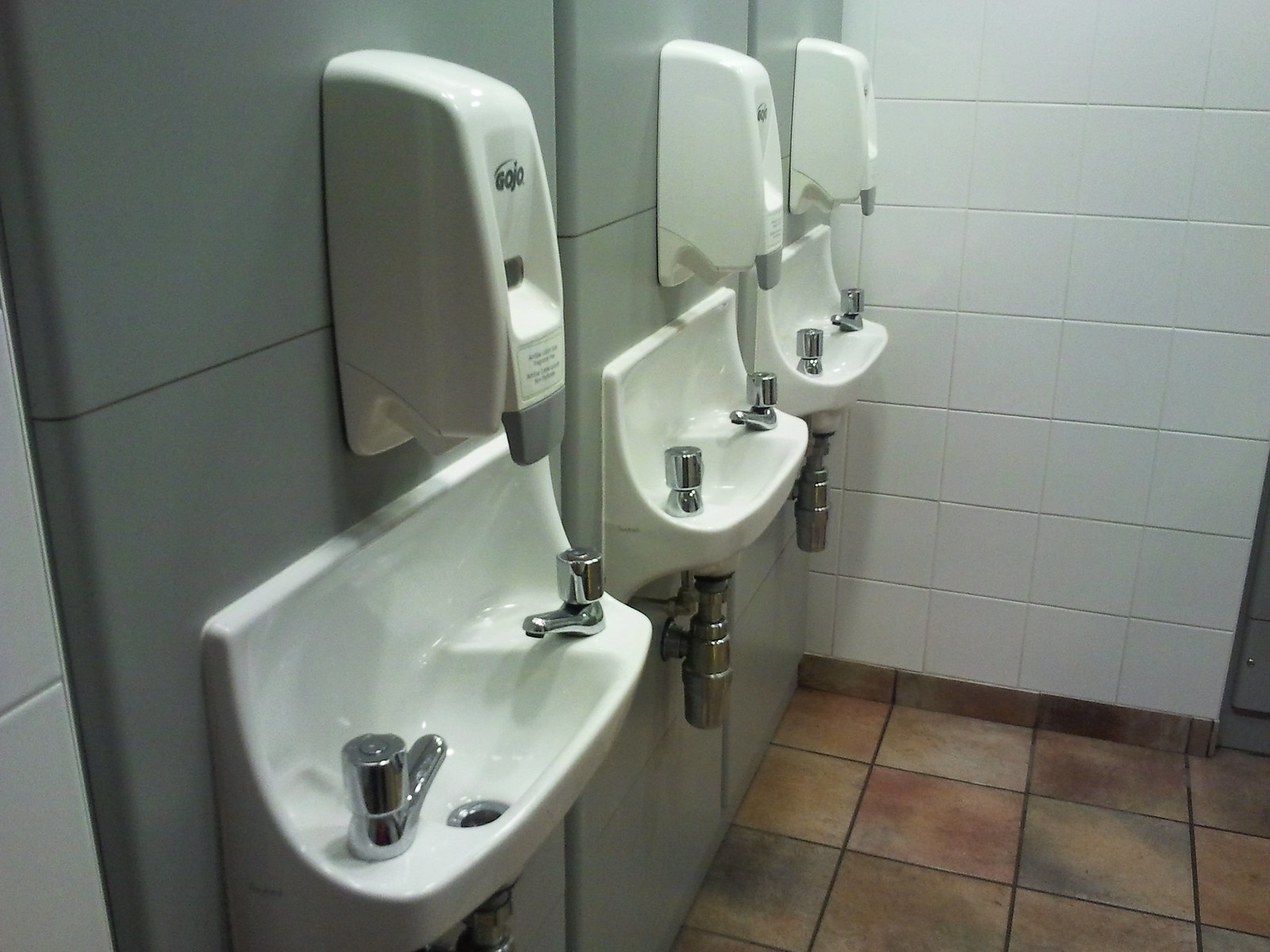The image depicts a public bathroom, likely from a school or restaurant, with distinctive features. The floor has a mottled, multicolored tile design, predominantly beige with hints of blue and red, creating a watercolor effect. The walls are primarily white tiled, but the wall behind the sinks and soap dispensers is gray. Centered in the image are three small, white porcelain sinks, each recessed only four to five inches from the wall. Above these sinks are white Gojo soap dispensers with gray push buttons and gray lettering. Each sink is equipped with silver faucets on either side and visible silver piping below. The bathrooms' compact sinks emphasize their functional design in a limited space.